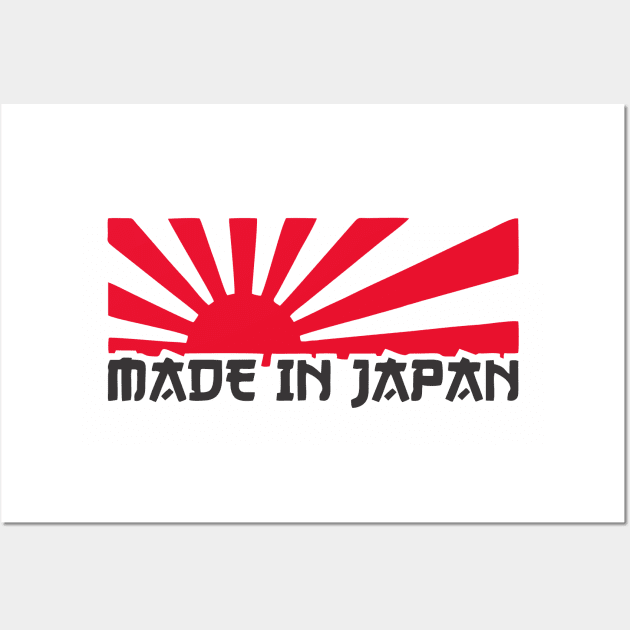The artwork features a central emblem known as the Japanese rising sun flag, set against a white backdrop that is further positioned on an off-white background. The rising sun emblem is vividly detailed, displaying nine red rays emanating from its center. Below this striking image, the text "Made in Japan" is prominently displayed in a modern, stylized English font that mimics Japanese calligraphy. The text features all capital letters with unique characteristics such as curved and marked letters, giving it a distinct, Japanese-inspired design.